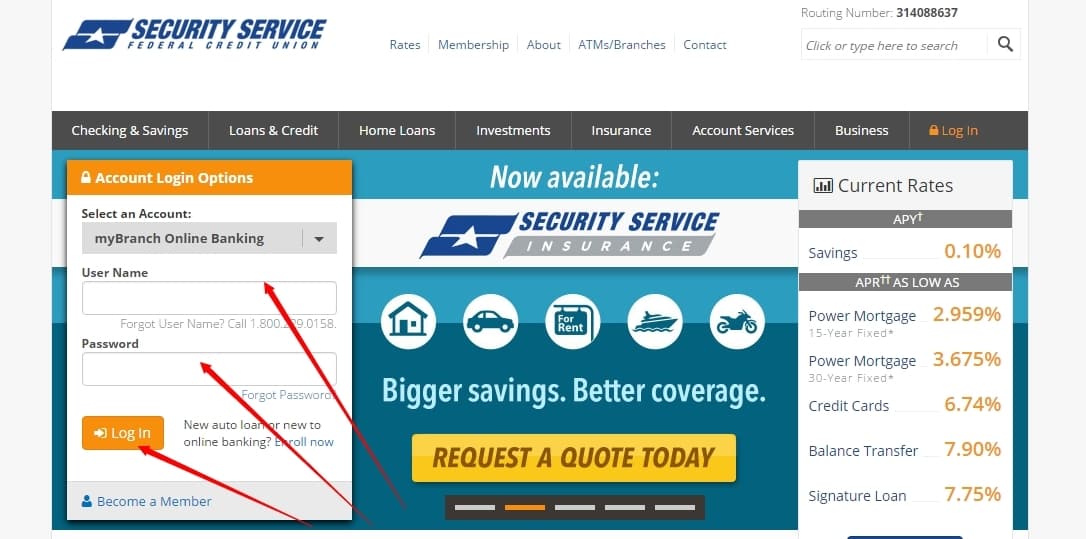The image captures a web page for Security Service Federal Credit Union. The page features two gray vertical bars on the left and right, each taking up about an eighth of the space. On the upper part of the white background, the text "Security Service Federal Credit Union" is written in blue. In the center, in black text, it states "Waits Membership or Ballot, ATM/Branches Contract."

The routing number, 314088637, is also displayed. There's a search box for users to type queries into. Various navigation buttons are present, each with a white background and text including: "Checking and Savings," "Loans and Credit," "Home Loans," "Investments," "Insurance," "Account Services," and "Business." An orange login button is also visible.

On the left side of the screen, there is a pop-up menu with a gradient background moving from baby blue to darker blue. The popup has "Account and Login Options" in white text on a yellow-orange background. Below, it displays fields for "My Branch Online Banking," "Username," and "Password," with a login button. Red arrows point to these fields to guide users through the login process.

A section titled "Available Now" promotes Security Services, with images of a house, car, "For Rent" sign, boat, and motorcycle. Accompanying text in white reads "Bigger Savings, Better Coverage," with a call-to-action "Request a Quote Today" highlighted in yellow.

On the right side of the page, current APYs are displayed as follows:
- Savings: 0.10%
- Powered Mortgage: 2.9%
- One: 3.6%
- Credit Cards: 6.7%
- Balance Transfer Chart: 7.9%
- Signature Loan: 7.5%

The overall design may suggest this screenshot was taken many years ago, given the notably higher financial terms compared to today's standards.